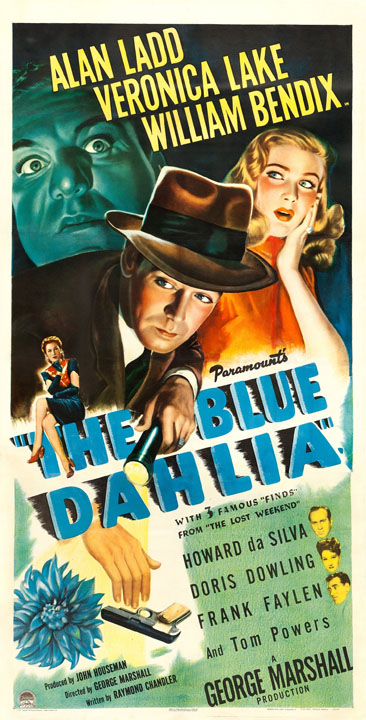This is a vintage movie poster for the film "The Blue Dahlia." The poster, rendered in a classic old movie style, is in portrait format and features painted illustrations of the main characters. At the top, the title "Paramount's The Blue Dahlia" is prominently displayed in blue text, stretching horizontally across the poster. Above the title, the leading stars Alan Ladd, Veronica Lake, and William Bendix are credited in bold yellow type against a dark background.

The central illustration portrays a detective, dressed in a brown suit and fedora, leaning forward with a flashlight, giving an investigative vibe reminiscent of the 1950s Hardy Boys style. The detective appears to be interacting with the title "The Blue Dahlia," adding a dynamic element to the poster.

Alongside the main detective figure, the poster includes smaller images of other characters, such as a woman who looks aghast, and a sinister-looking individual with green skin, hinting at a thriller or mystery genre. The bottom of the poster provides additional text, including other cast members' names—Howard Da Silva, Doris Dowling, Frank Phelan, and Tom Powers—alongside production details, noting it as a George Marshall production. The lower left also features a Blue Dahlia flyer and a gun, adding to the movie's suspenseful atmosphere.